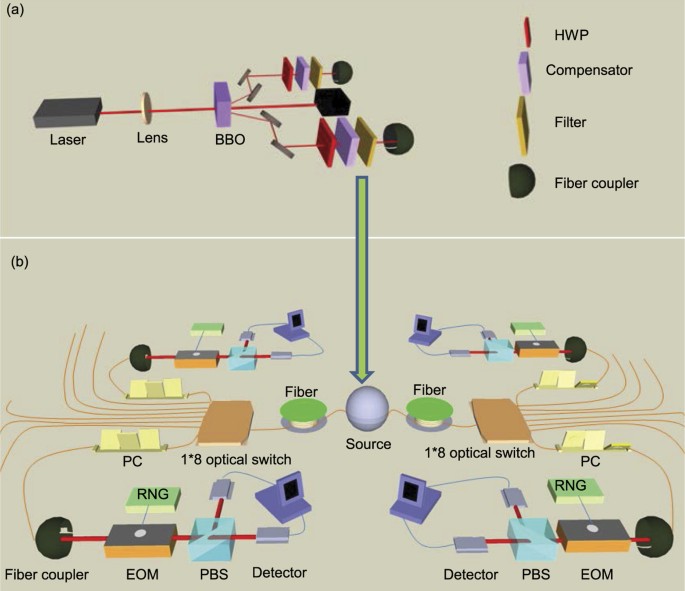This image is a detailed diagram of an electronic device, split into two panels labeled A (top) and B (bottom). Panel A, occupying about two-fifths of the image, features interconnected components including a laser, lens, and BBO, all linked by red lines that possibly indicate wiring. A legend to the right specifies that red denotes HWP, purple is for compensator, yellow represents filter, and black indicates fiber coupler. A prominent green arrow with a bluish-purple outline points downward from Panel A to Panel B, signifying the direction of flow or connection.

Panel B, which takes up the remaining three-fifths of the image, includes a variety of labeled components connected by various colored lines. The labels here include fiber, source, a 1-to-8 optical switch, PC, RNG, EOM, PBS, and detector. Both panels are heavily integrated with numerous wires connecting all these devices, indicating a complex network of electronic or optical components.